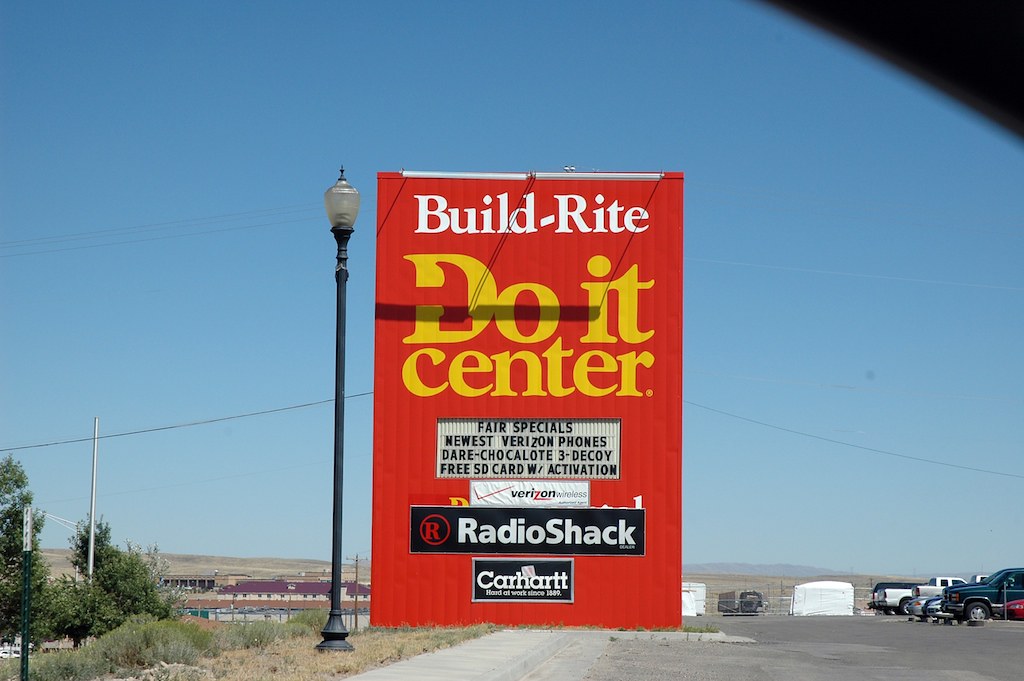This photograph features a large, prominently displayed sign with multiple advertisements. The top section of the sign reads "Build Rite," with the word "Rite" intentionally misspelled as "R-I-T-E." Below it, another large sign displays "Do It Center." The marquee board underneath lists various fair specials, including "Newest Verizon Phones," "Dare Chocolote" (chocolate misspelled as "C-H-O-C-A-L-O-T-E"), and "Free SD Card with Activation." Additional advertisements for “Radio Shack” and “Carhartt” are affixed to the side of the main sign.

A tall lamppost stands adjacent to the sign, nearly matching its height. The foreground reveals a parking lot filled with numerous pickup trucks. In the background, the arid landscape suggests a desert environment, with minimal greenery. The sky above is a clear blue, with no clouds in sight.